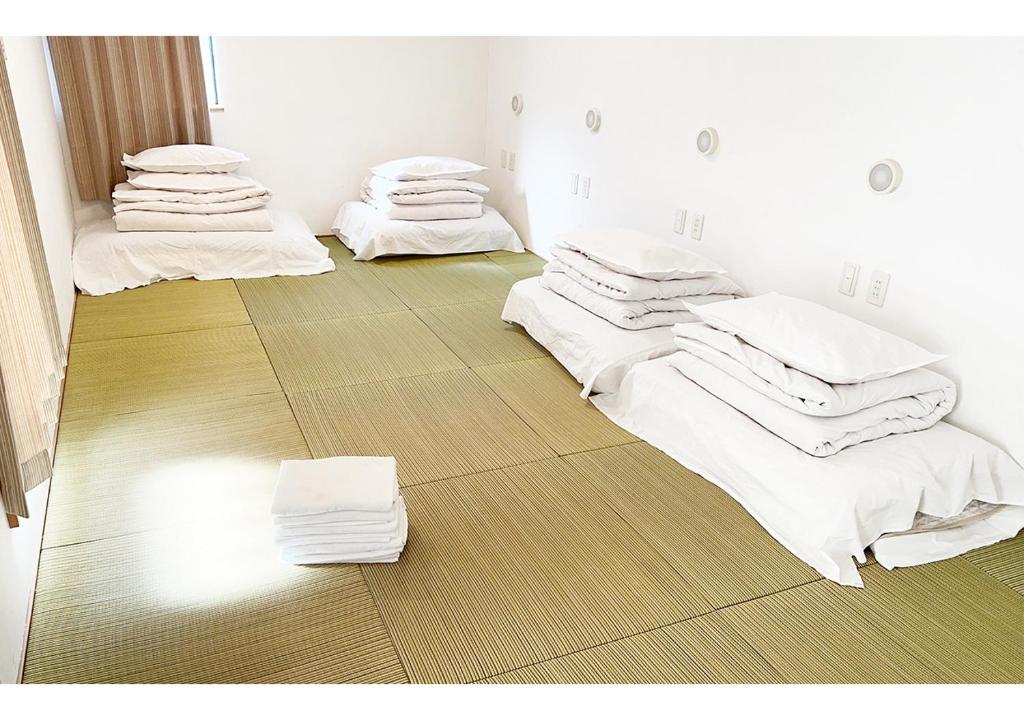The image depicts a small, rectangular, white-walled room with soft-textured, greenish square tiles that resemble strands of bamboo. The room is fitted with several outlets and lights, evenly distributed in four rows along the right wall. On the left side of the room, there's a patch of bright white sunlight highlighting stacks of neatly arranged white kitchen cloths in the middle of the floor. Against the walls on both the left and right sides, there are piles of bedding, including blankets, sheets, and pillows. Light brown curtains adorn the windows, reinforcing the room's indoor setting. Scattered around the room are a few mattresses with white covers, adding to the impression that this space could be used for sleeping or resting.